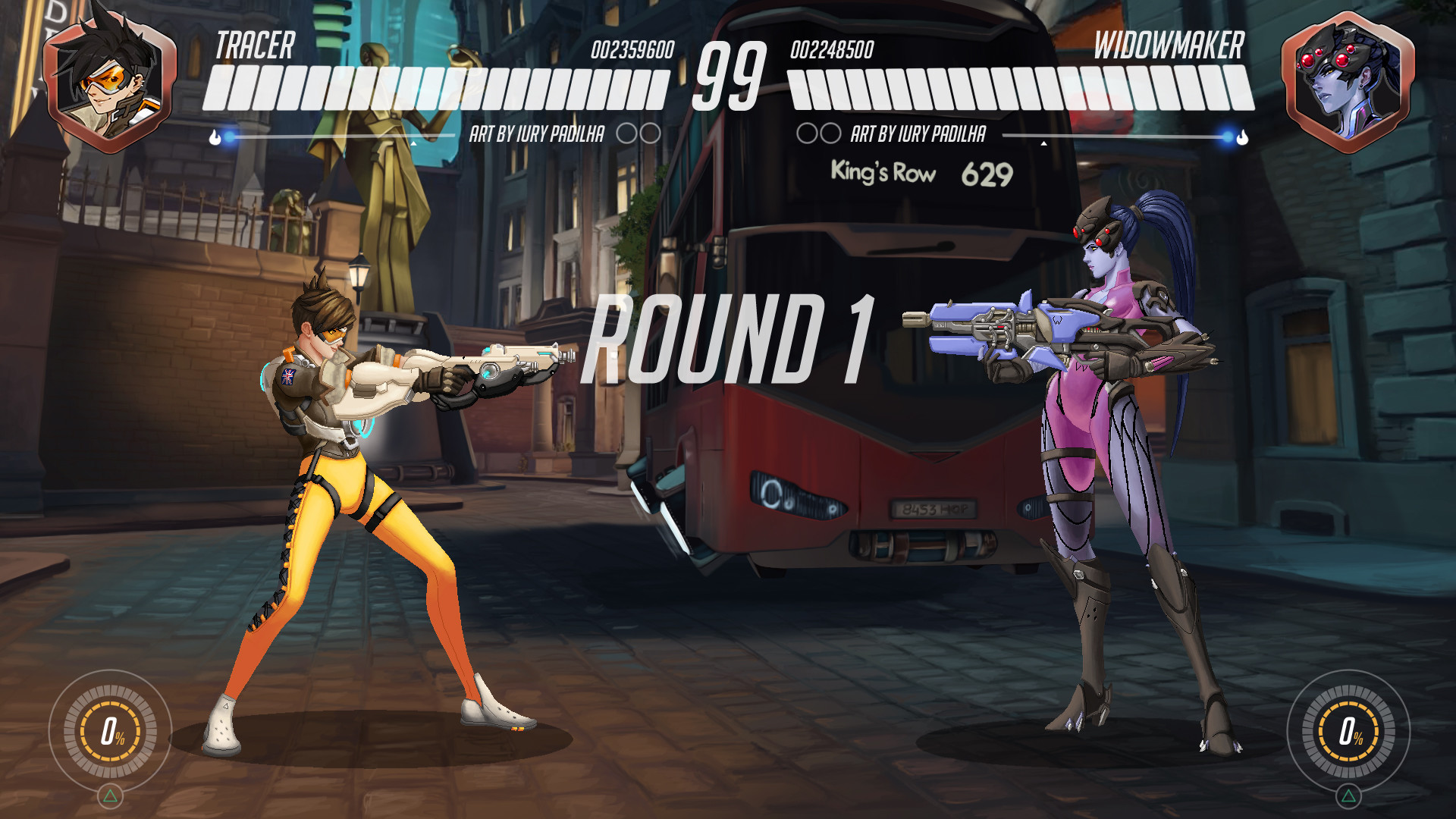This image, likely a screenshot from a video game, depicts two female characters poised for combat. In the center of the screen, "Round One" is prominently displayed in white text, above a timer set at 99. On the left is Tracer, wearing yellow leggings, white shoes, a mostly gray top, and yellow sunglasses. She holds a large gun pointed at her opponent. Tracer appears more human in comparison to the character on the right, Widowmaker. Widowmaker has a distinctly non-human appearance with bluish skin and a long blue ponytail. She is dressed in a pink, gray, and lavender outfit, with blue and black leggings, and wields a large blue and gray gun. Behind the characters, a cobblestone street can be seen, along with buildings, a statue, and a double-decker bus marked "King's Row 629." At the top of the screen, the names Tracer and Widowmaker are displayed along with their portraits in hexagonal frames, indicating their health scores at 99 each, both at full health.